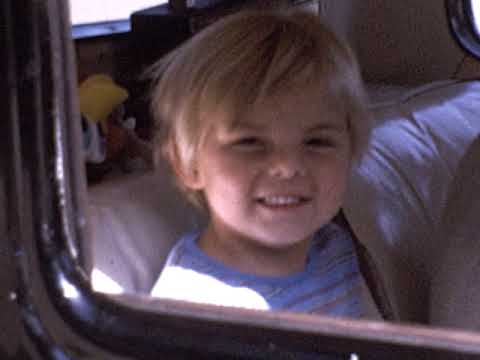A cheerful young boy, around five years old, with short, somewhat messy blonde hair, is captured smiling directly at the camera from the backseat of a vehicle. His fair skin and bright demeanor stand out against the slightly fuzzy background. The boy is wearing a blue striped t-shirt, which features both blue and red stripes. He is seated on a beige-colored seat, likely within a darker-colored vehicle. The image, taken through a window, shows some indistinct objects behind his head, possibly in the trunk space, including a yellow toy and various other items. To the right of the boy, only an arm and shoulder of another person are visible, hinting at someone else in the vehicle, perhaps the driver. Despite the blurriness, the focus is clearly on the boy's joyous expression, highlighting the innocence and delight of a moment spent in transit.